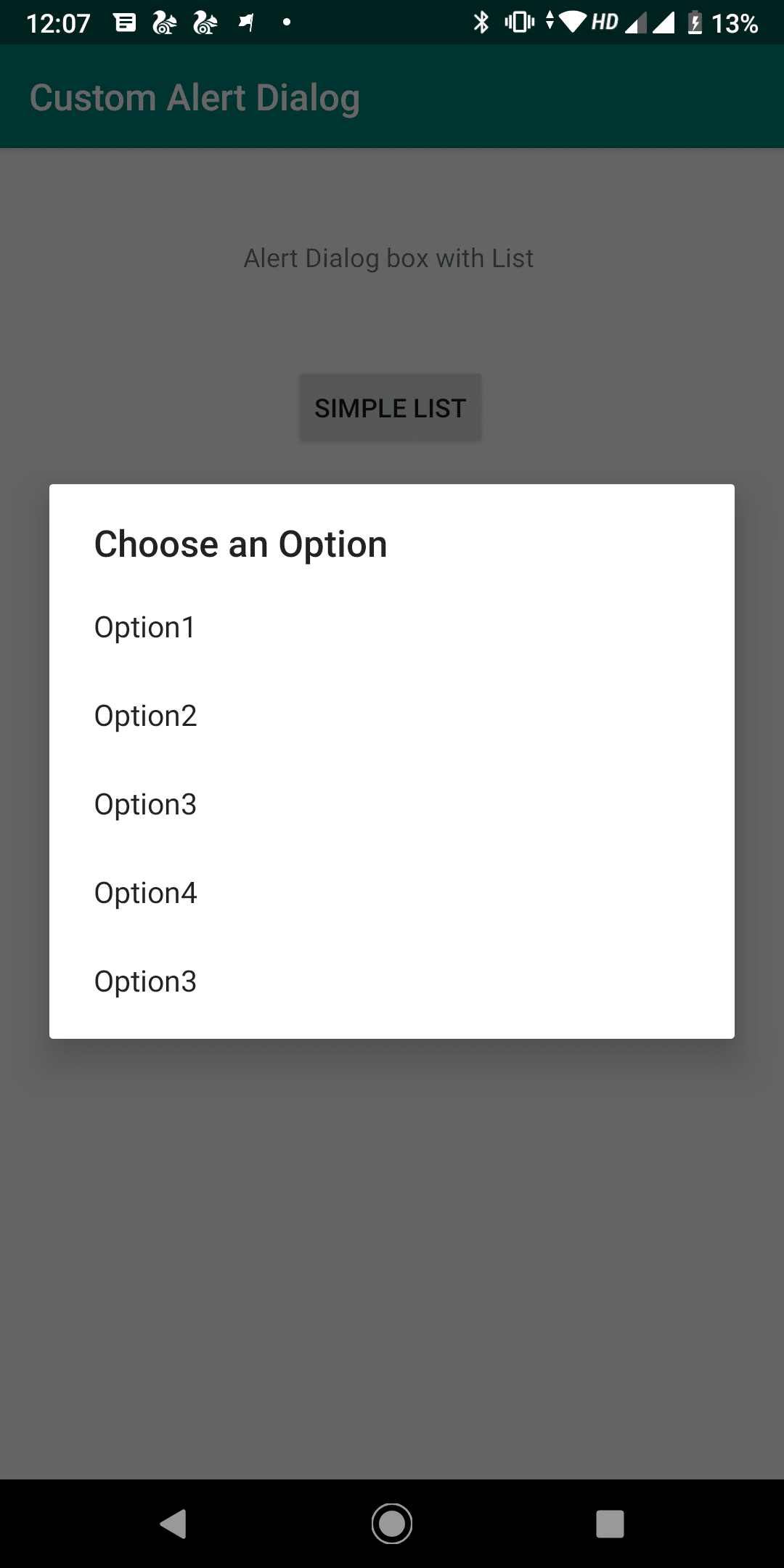The image is a vertically-oriented screenshot that appears to be taken from a smartphone, possibly an iPhone or Android. At the very top of the image, a thin black bar displays the standard smartphone status icons in white. On the upper left of this bar, the time reads "12:07," followed by symbols including a square with white bars, two icons resembling squirrels, a flag symbol, a white dot, and a "B" icon. To the far right, there are additional symbols, including a battery icon, two triangles stacked vertically (one pointing up, the other down), a white Wi-Fi symbol, and the letters "HD." Additionally, there are two indicators of signal strength—one showing three bars and the other showing full bars. Next to them is a Facebook icon and "13%" indicating battery percentage.

Below the black bar is a green bar with white text that reads "custom alert dialog." The primary section of the image is dominated by a large white box that appears to overlay the screen, causing the background to be grayed out. Inside this white box, in the upper left corner, black text reads "Choose an option." Below this, five selectable options are listed vertically as "Option 1, Option 2, Option 3, Option 4," and again "Option 3."

In the background, partially obscured by the white box, there is some black text at the top saying "alert dialog box with list." Below this text, there is a clickable gray box labeled "simple list," which might be responsible for displaying the large white options box.

At the very bottom of the image, a prominent black bar contains several gray symbols. On the left side of this bar are play and stop buttons, with a gray circle in the center and surrounding black edges. On the lower right side, there is a gray square icon.